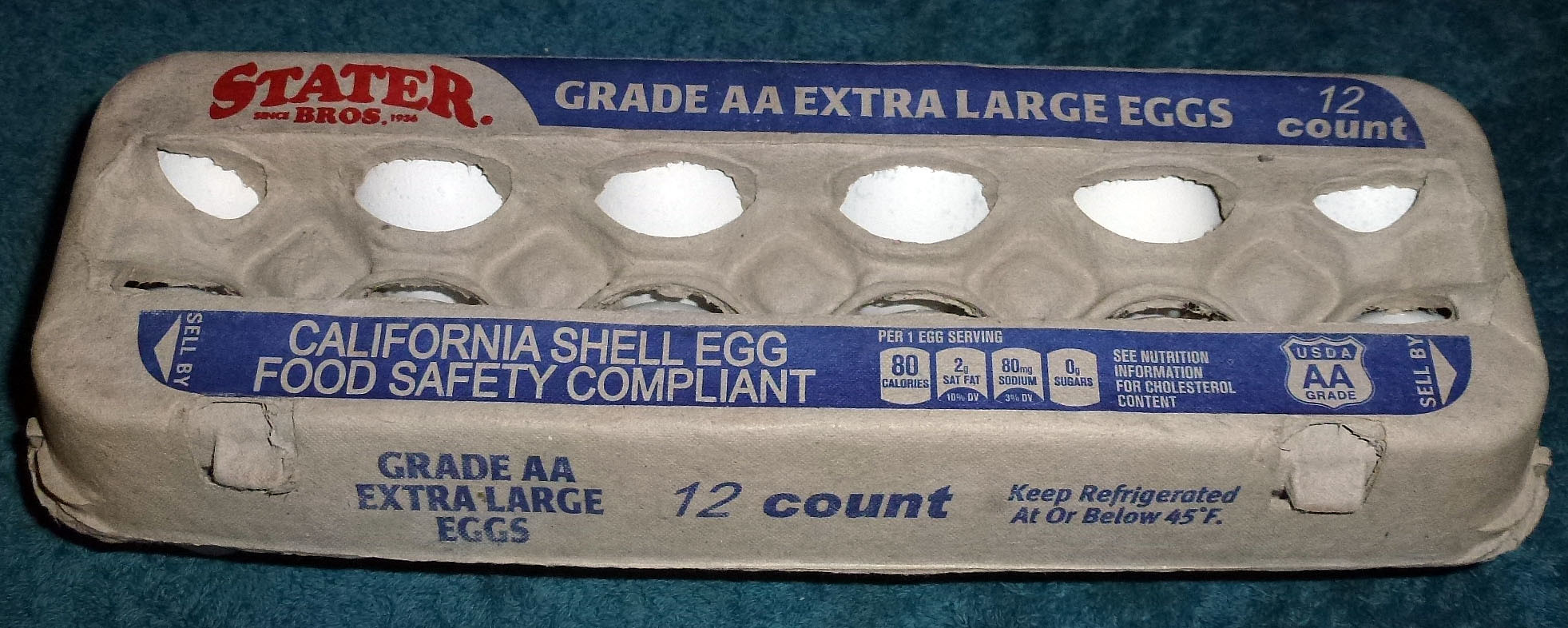This image displays a grey cardboard carton of Stater Brothers eggs, featuring a vibrant red "Statler Brothers" logo on the top left corner. The carton holds a dozen Grade AA extra-large eggs, which are visible through the cutouts on the top of the box. The blue branding details indicate the eggs are California Shell Egg Food Safety Compliant and must be kept refrigerated at or below 45 degrees Fahrenheit. Nutritional information is prominently displayed, noting that each egg contains 80 calories, 2% saturated fat, 100 mg of sodium, and 0 sugars. The carton, from a brand established in 1934, adheres to USDA standards providing a clear view of six white eggs from the aerial perspective.